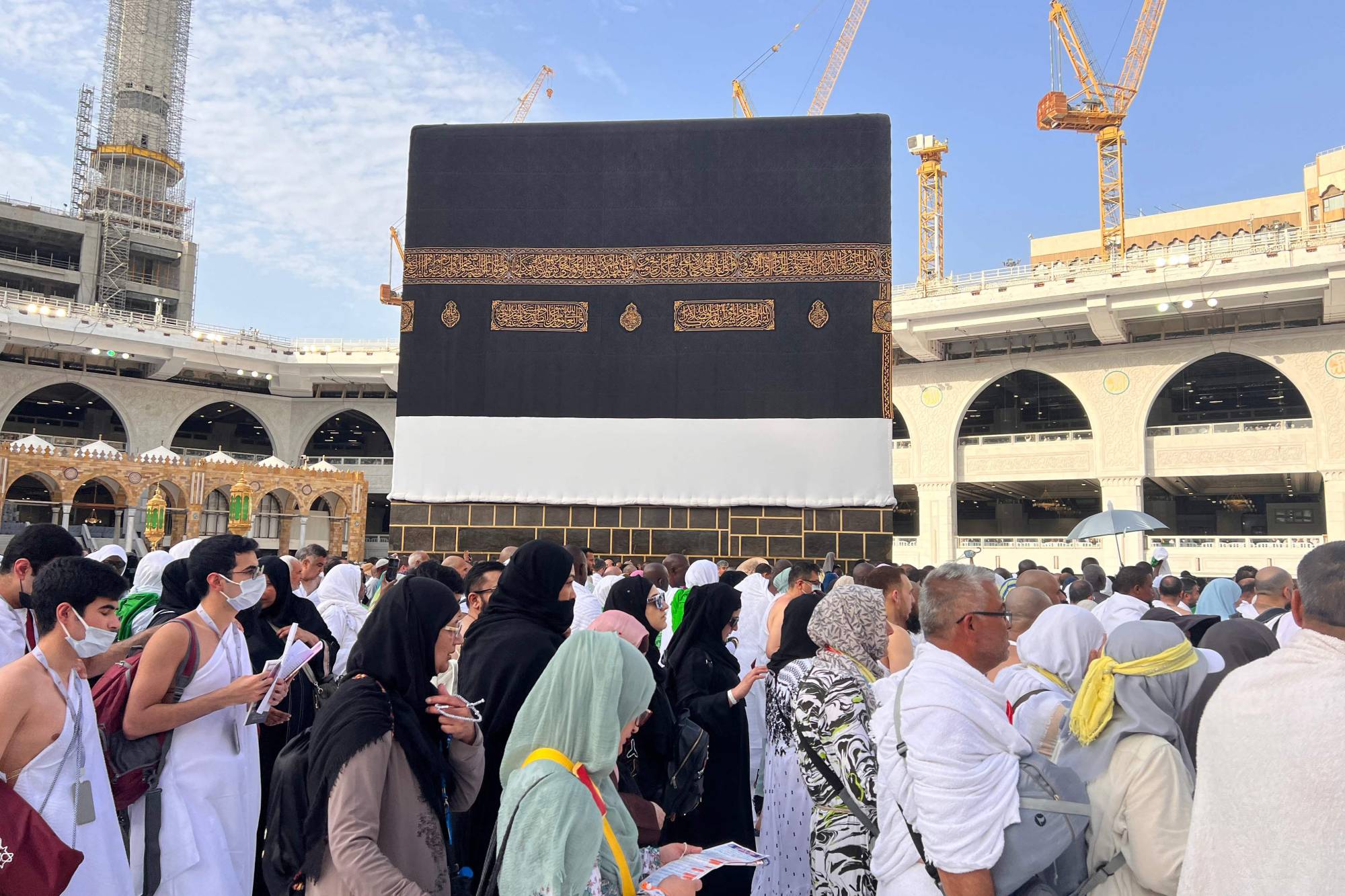This photo, reminiscent of a travel magazine shot, captures a bustling crowd of people walking around the Kaaba in the holy city of Mecca, Saudi Arabia, during the day. The Kaaba, a cube-shaped structure draped in a black tapestry, stands as the focal point within an open area encircled by worshippers. The individuals in the crowd are seen moving from left to right, with many wearing headdresses and face masks, indicative of the diverse assembly of men and women. Some men are dressed in white toga-like garments, while others sport regular long-sleeve shirts. Numerous people carry handbags and backpacks, often with tags hanging from lanyards around their necks, suggesting a traveling pilgrimage. The background reveals a multi-level structure adorned with archways and significant construction activity marked by several yellow cranes, emphasizing ongoing development in the surrounding area. The scene is one of vibrant movement and deep spiritual significance.